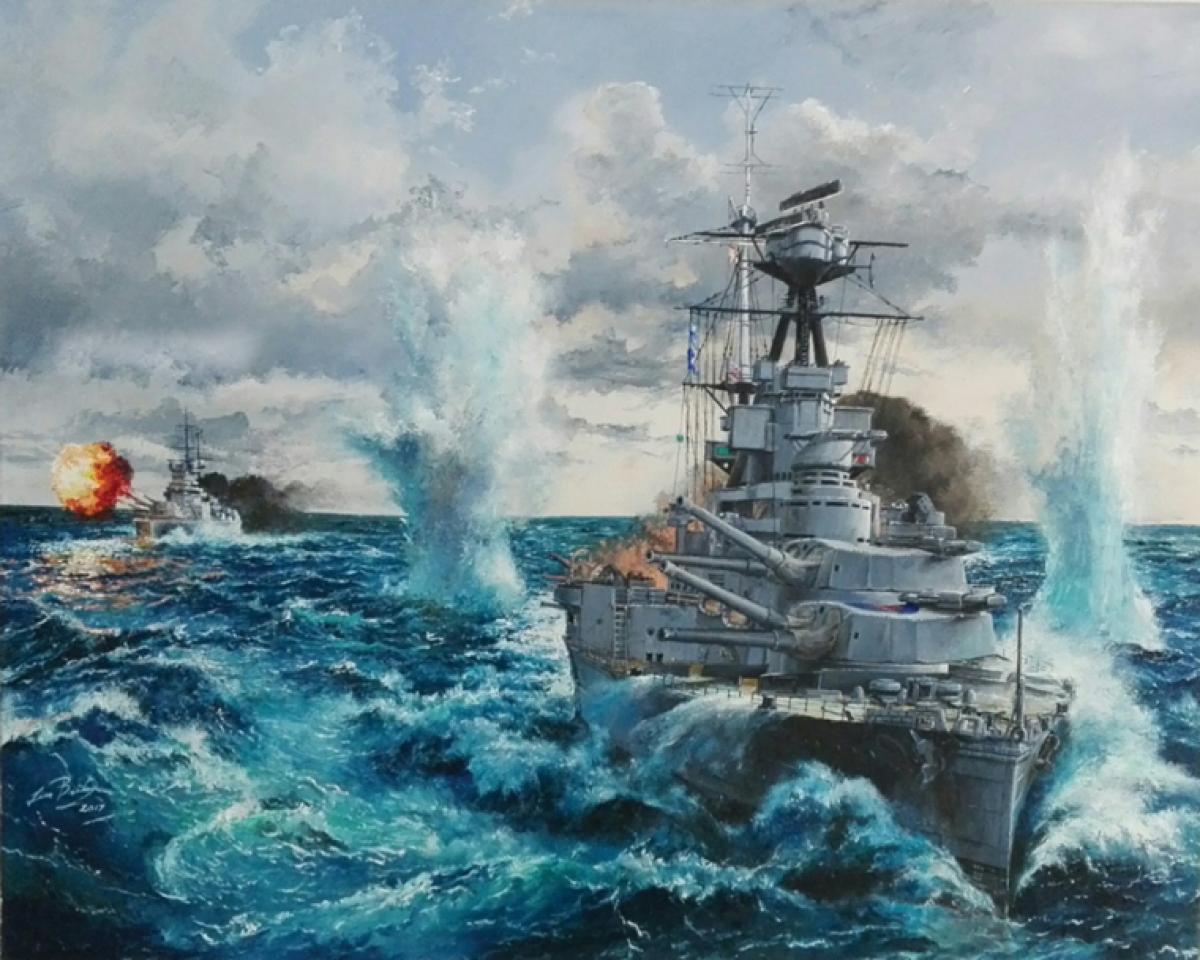The painting powerfully captures a dramatic World War II naval battle at sea, dominated by a large, modern battleship in the foreground on the right. This battleship, equipped with imposing 16-inch guns and likely featuring sonar, is charging toward the viewer's perspective, cutting through the deep blue, choppy ocean. Its wake disrupts the turbulent waves, adding to the sense of dynamic movement. Surrounding the battleship are several water splashes, indicative of enemy shells hitting nearby, while smoke billows from its rear. To the left and further back, a smaller cruiser is depicted in the act of firing its cannon, with a vivid explosion of red and yellow fire bursting from the muzzle. This cruiser also has black smoke trailing from its back, suggesting that it has sustained hits. The sea, agitated both by the high-speed maneuvers of the ships and the impacts of explosions, is matched by a stormy sky above, filled with pale blue tones and ominous clouds, completing the intense and chaotic scene of warfare.